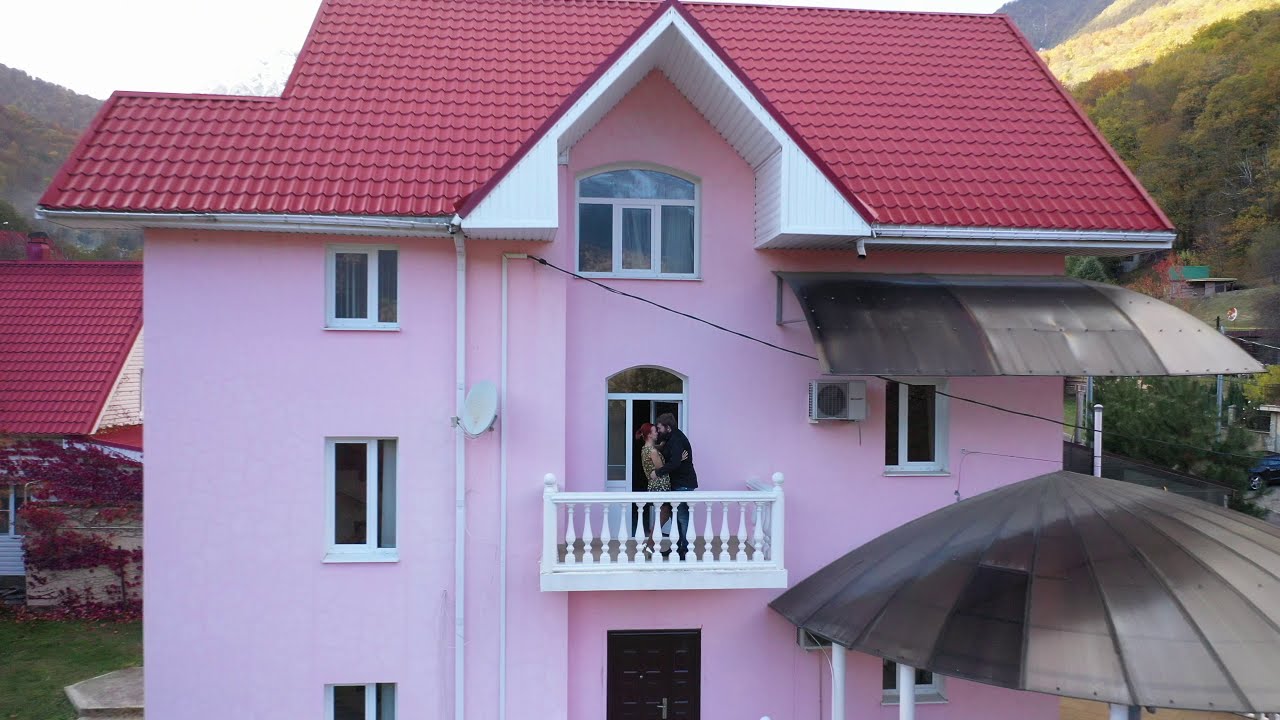This photograph captures a striking three-story pink house with a red-tiled roof. Prominently on the second story, a white balcony hosts a couple, seemingly in an affectionate embrace or kiss. To the left of the couple, a satellite dish is fixed to the building. On the right side of the structure, a couple of dark-colored awnings extend over some windows. The building's immediate surroundings feature several other houses and structures, all nestled in a lush valley enclosed by green hills. Behind the house, verdant inclines rise steeply, dotted with trees. A sliver of a white, blurry sky is visible at the top edges of the image. The couple’s attire is partially distinguishable; the man appears to be in a black suit, while the woman seems to be wearing a yellow and black dress.